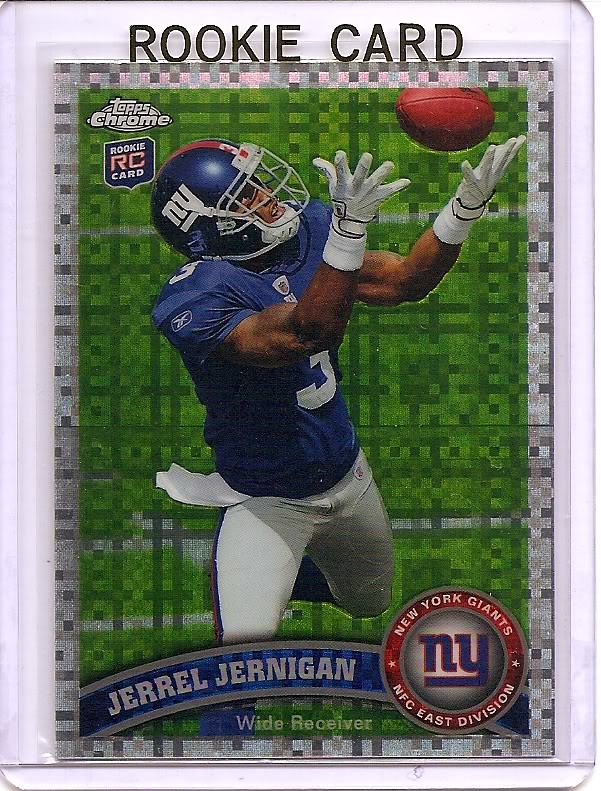This image showcases a meticulously preserved football card encased in plastic, known for its iconic designation as a "rookie card." The card features a white border with "rookie card" emblazoned in black at the top. At its heart is an action shot of football player Jarrell Jernigan, a wide receiver for the New York Giants. Jernigan is captured mid-air, lunging forward to catch a football. He dons a blue jersey with the number 3, a blue helmet with white trim, white football pants, and strikingly large white gloves reminiscent of Mickey Mouse gloves. The background is a green, pixelated rendition of a football field complete with white lines, giving the impression of in-game action. At the bottom, a blue, arched banner bears Jernigan’s name in white text. To the right, a red-outlined circle prominently features the New York Giants logo along with "NY," "NFC East Division," and "New York Giants." The card also bears the "Topps Chrome" brand insignia discreetly placed, adding a layer of authenticity.